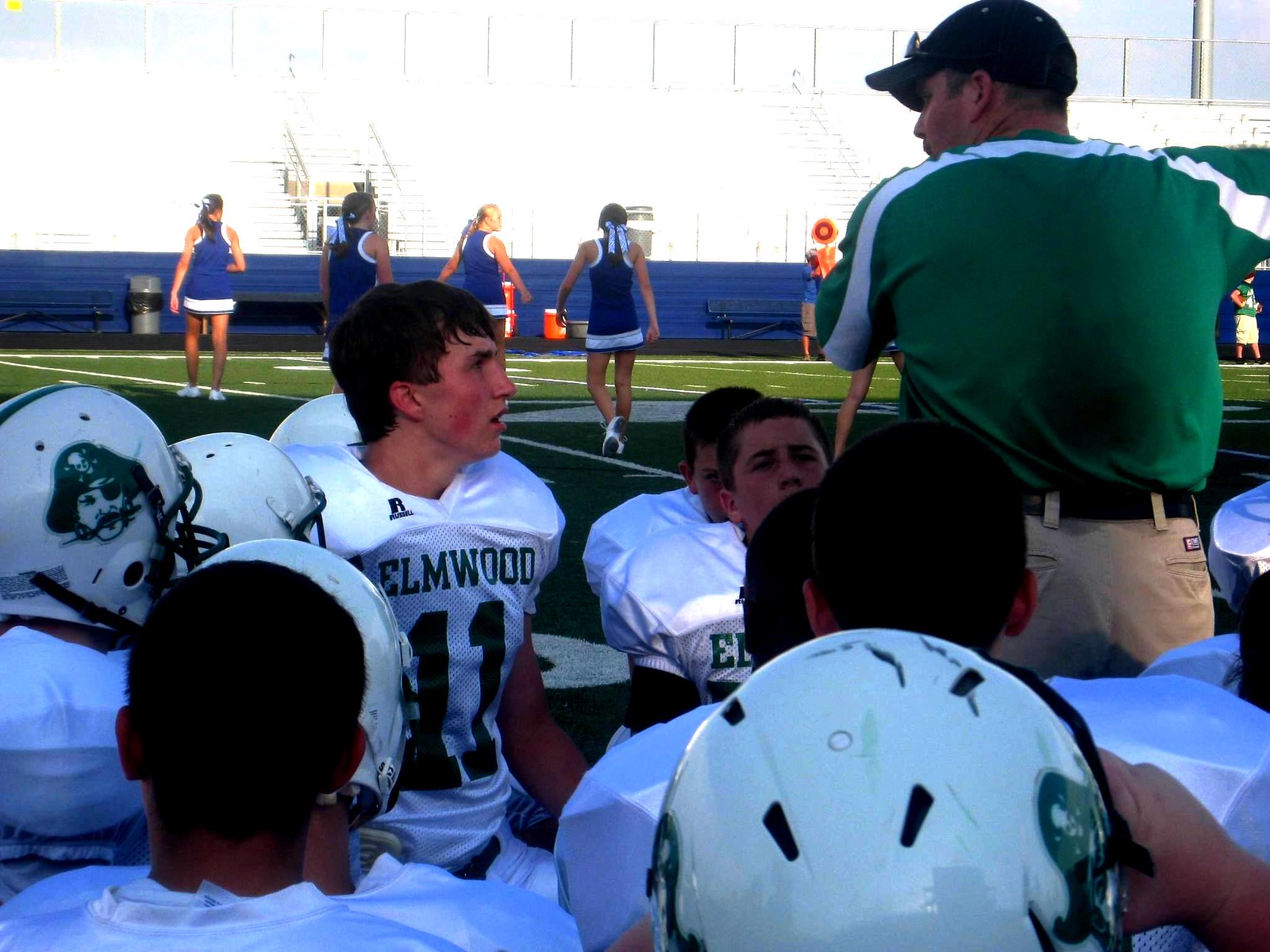In the foreground of this image, a high school football team named Elmwood is gathered around their coach, who appears to be giving a motivational speech. The coach, facing away from the camera, is dressed in a green and white striped polo shirt, a black hat, and khaki shorts. The players, some donning their helmets and others not, wear green and white jerseys with the name "Elmwood" and display a green pirate logo on their helmets. Surrounding them are white lines marked on the grass football field, indicating yardage. In the background, a group of cheerleaders are dressed in blue and white uniform dresses with white shoes, adding vibrant energy to the scene. Behind them, blue bleachers stand against a bright, clear sky, bordered by fences and signage that hint at a lively, well-attended event. The whole composition suggests a bustling and spirited atmosphere, likely before or after an intense game.